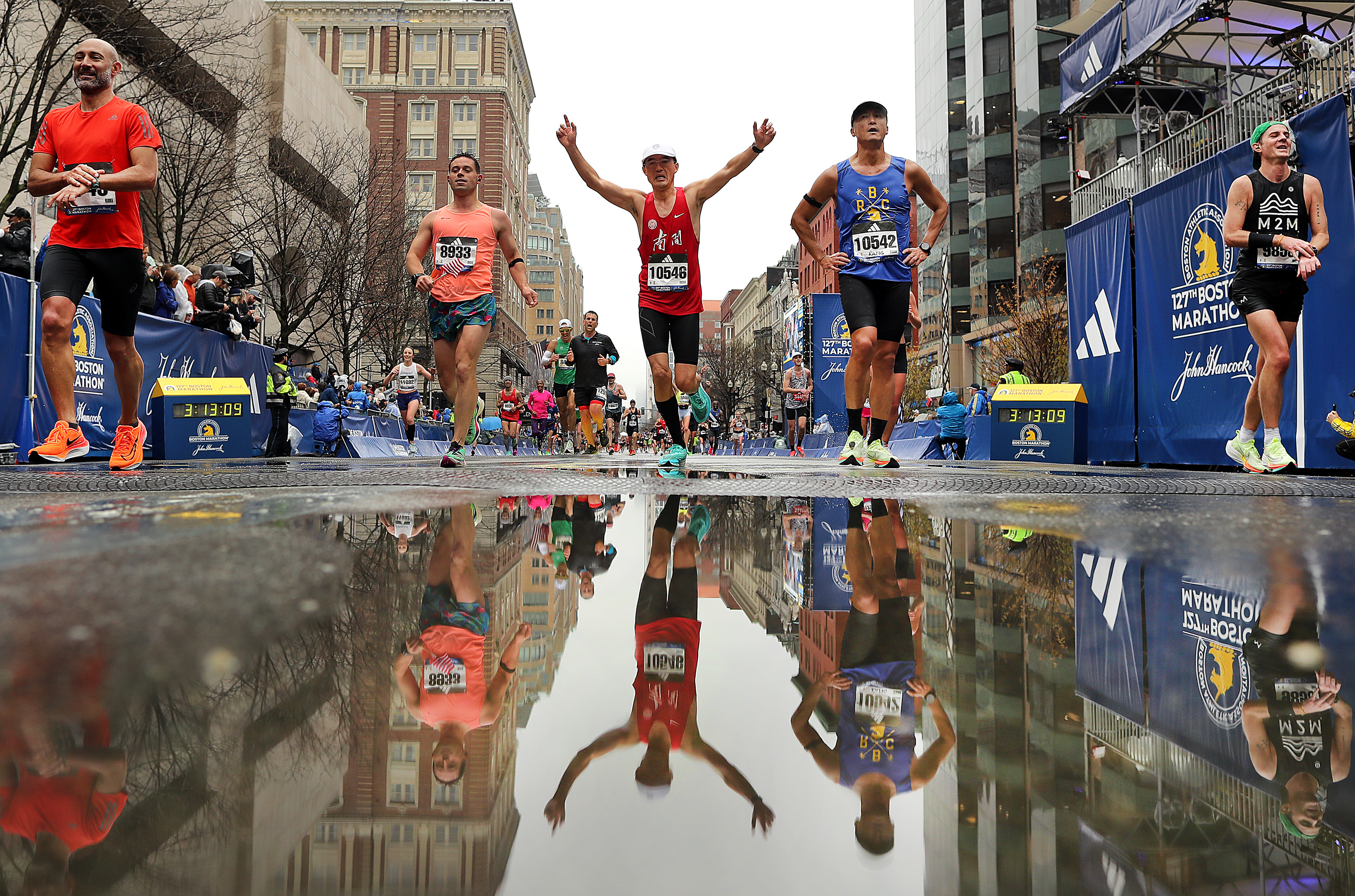This captivating color photograph, taken from a low angle, beautifully captures the energy and excitement of the 127th Boston Marathon. The image showcases a group of five marathon runners nearing the finish line on a city street lined with tall buildings. These runners are prominently reflected in a large, pristine puddle of water in the foreground, creating a stunning mirror effect that doubles the lively scene.

The central runner, exuberant with both arms raised in celebration, wears a sleeveless red jersey, aqua-colored shoes, and sports a race number on his chest. To his right, another runner in a blue sleeveless shirt, black pants, and a white cap appears exhausted with hands on hips. Flanking the central runner on the left is an athlete in a peach-colored shirt and blue patterned shorts, while the far-right runner dons black attire, white shoes, and a green cap. An older runner in a red t-shirt and black shorts, wearing orange shoes, completes this front group, displaying remarkable endurance with a less fatigued demeanor.

In the background, a multitude of runners continues the race, creating a dynamic vanishing point against the backdrop of brick, brownstone, and concrete buildings. Spectators can be seen cheering from the sidelines, adding to the event's festive atmosphere. Large banners announcing "127th Boston Marathon" and sponsored by John Hancock, along with an Adidas logo, hang prominently along the barriers. The official marathon clock reads 3:13:09, indicating a commendable finishing time. The hazy sky hints at the earlier rain shower that left the reflective puddle, enhancing the photograph's artistic composition and making this image a memorable representation of the marathon's spirit and resilience.